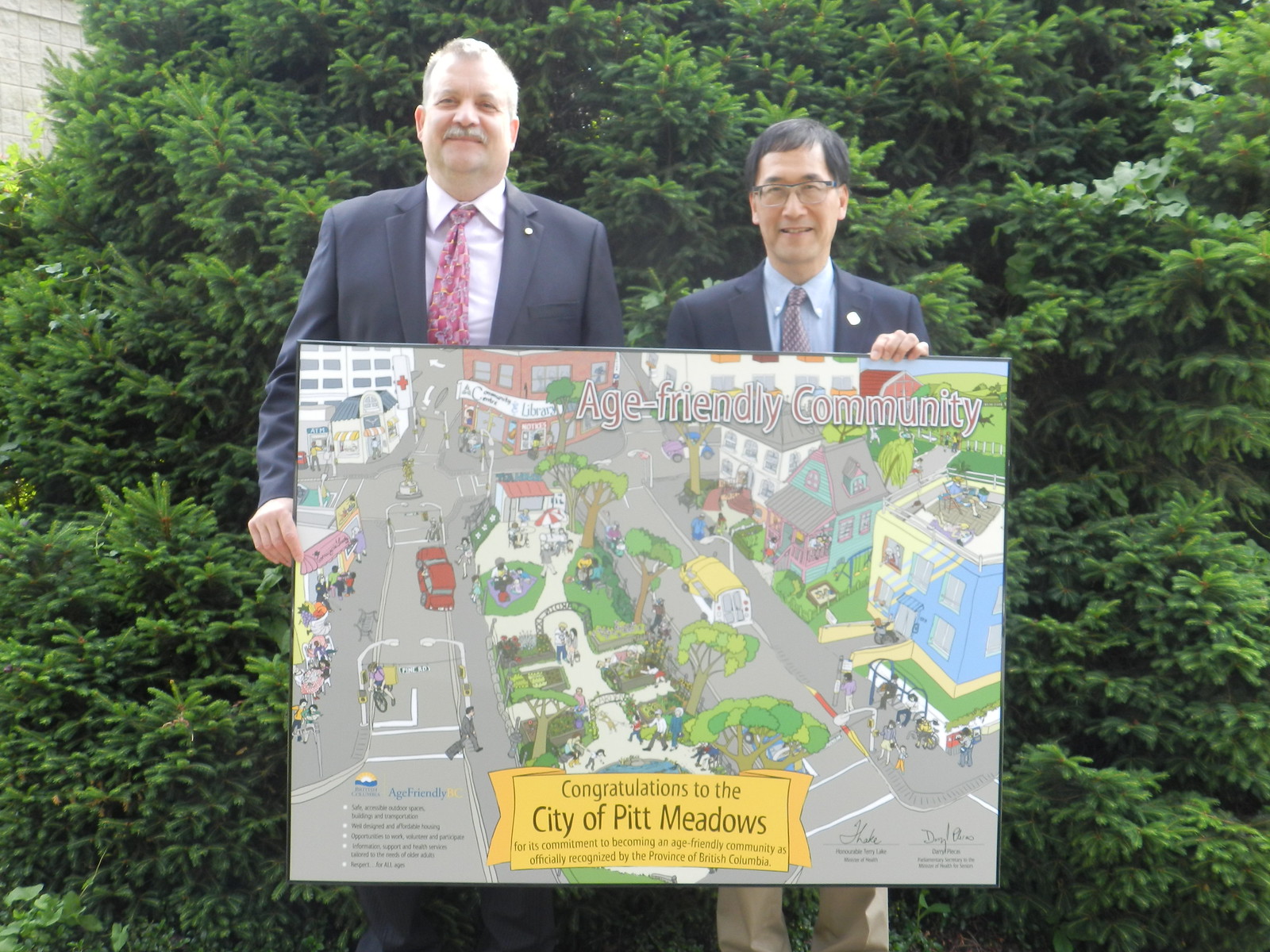In this somewhat faded, full-color outdoor photograph taken during the day, two men pose in front of a backdrop dominated by lush green evergreen trees. The man on the left is an older, taller Caucasian with short gray hair and a white mustache, dressed in a blue suit, light purple shirt, and a pink tie. The man on the right is an Asian gentleman with dark hair, wearing glasses, a blue suit, a blue shirt, and a darker purple tie. Together, they hold a colorful poster that appears to feature artwork typical of a children's book. This poster illustrates a vibrant town complete with houses, people of all ages, cars, streets, and various community amenities like parks, stores, a library, and a pharmacy. Prominently displayed on the poster is the phrase "Age-Friendly Community" in the upper right, while a yellow ribbon at the bottom declares, "Congratulations to the City of Pitt Meadows for its commitment to becoming an age-friendly community, as officially recognized by the province of British Columbia."